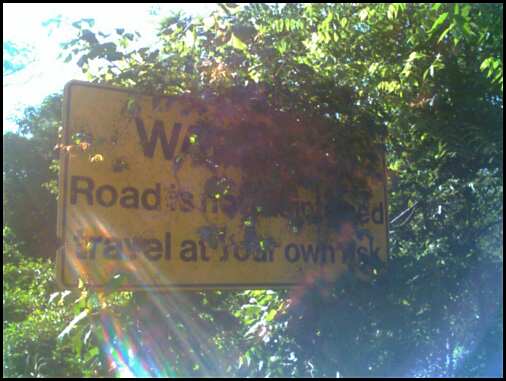This photograph captures a large, yellow road sign with a black border, largely obscured by a thick growth of vines, leaves, and moss. While the sign is somewhat blurry and partially distorted by sunlight filtering through the trees, key portions of its warning message can still be deciphered. The top line prominently displays "WA," likely short for "WARNING." Below, partially covered by foliage, it reads "road is not completed," and at the bottom, it cautions "travel at your own risk." The scene is bathed in natural light, with sun rays piercing through the dense tree cover in the top left corner, casting a glow across the verdant surroundings. The combination of foliage and tree coverage enveloping the sign indicates a scenic yet potentially hazardous unfinished road.